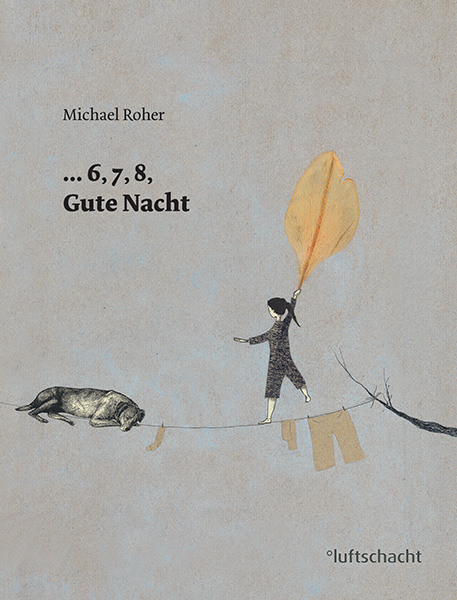The book cover is a vertical rectangle with a background blending gray and sepia tones. In the upper left corner, the text "Michael Roher" appears in black, followed by an ellipsis and the numbers 6, 7, 8, then "Guttnacht" in bold black letters. This likely indicates the author and title of the book. Centrally featured is a whimsical illustration: a brown and white dog lies on its left side, legs facing the viewer, head resting on its arm. A clothesline stretches across the center, anchored to a tree branch on the right. Hanging from the line are khaki pants and socks, while a girl in a black spotted outfit balances on the line, holding an oversized orange-brown leaf like a parasol. In the lower right corner, the word "Luftschacht" is displayed in black text.